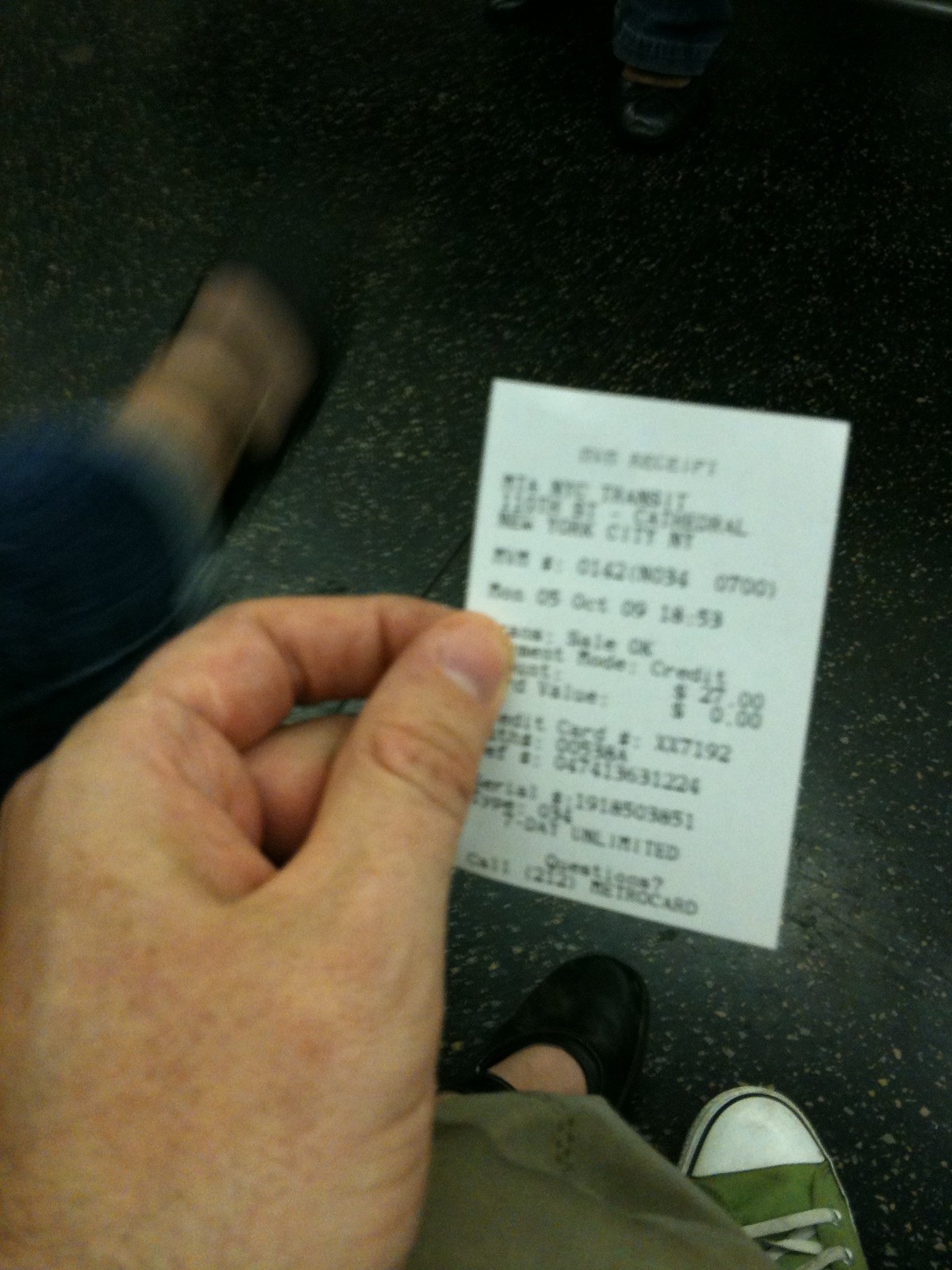In this vertical image, a human left hand with a medium skin tone is prominently featured holding a white receipt. The top of the receipt reads "RECEIPT" in large black text, followed by "NYC Transit." Below this are various numbers and letters, including a prominent "$27." At the very bottom of the receipt, it says "Questions" in black text, followed by "Call 212 MetroCard" on the line underneath. 

The background showcases a black floor adorned with white specks. The individual holding the receipt is wearing an olive green Converse-type shoe, partially visible, along with matching olive green pants. To the left of this person, a blurry leg clad in blue jeans and black shoes with two straps over the top is visible, indicating a right leg. Near the bottom center of the image, the matching shoe to the olive green one is discernible next to the other person's black strapped shoe.